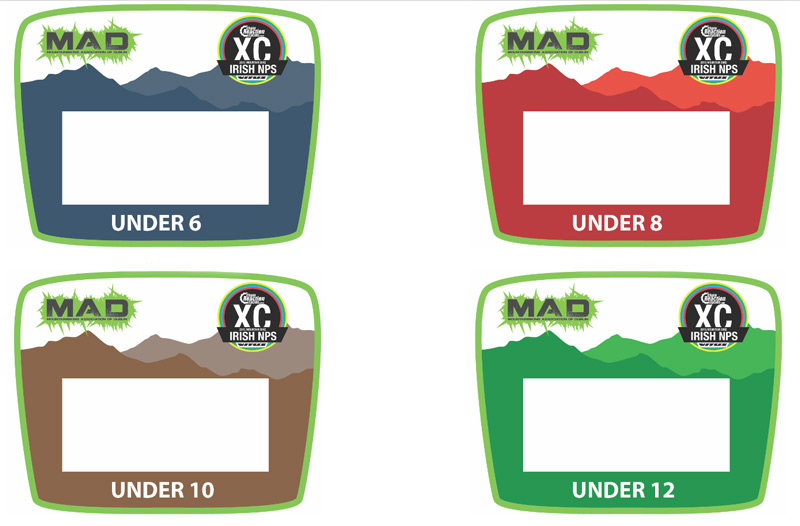The image features a white background with four distinct rectangular designs, each representing different age groups, possibly for a children's event or competition. Each design is color-coded: blue for "Under 6," red for "Under 8," brown for "Under 10," and green for "Under 12." In the top left corner of each rectangle, the acronym "MAD" is prominently displayed, likely indicating the sponsor. The top right corner features the text "XC Irish NPS" in black. Each design also includes a white rectangular space, potentially for writing a name or adding a picture, reinforcing the idea that these might be badges or labels for kids to indicate their age group.